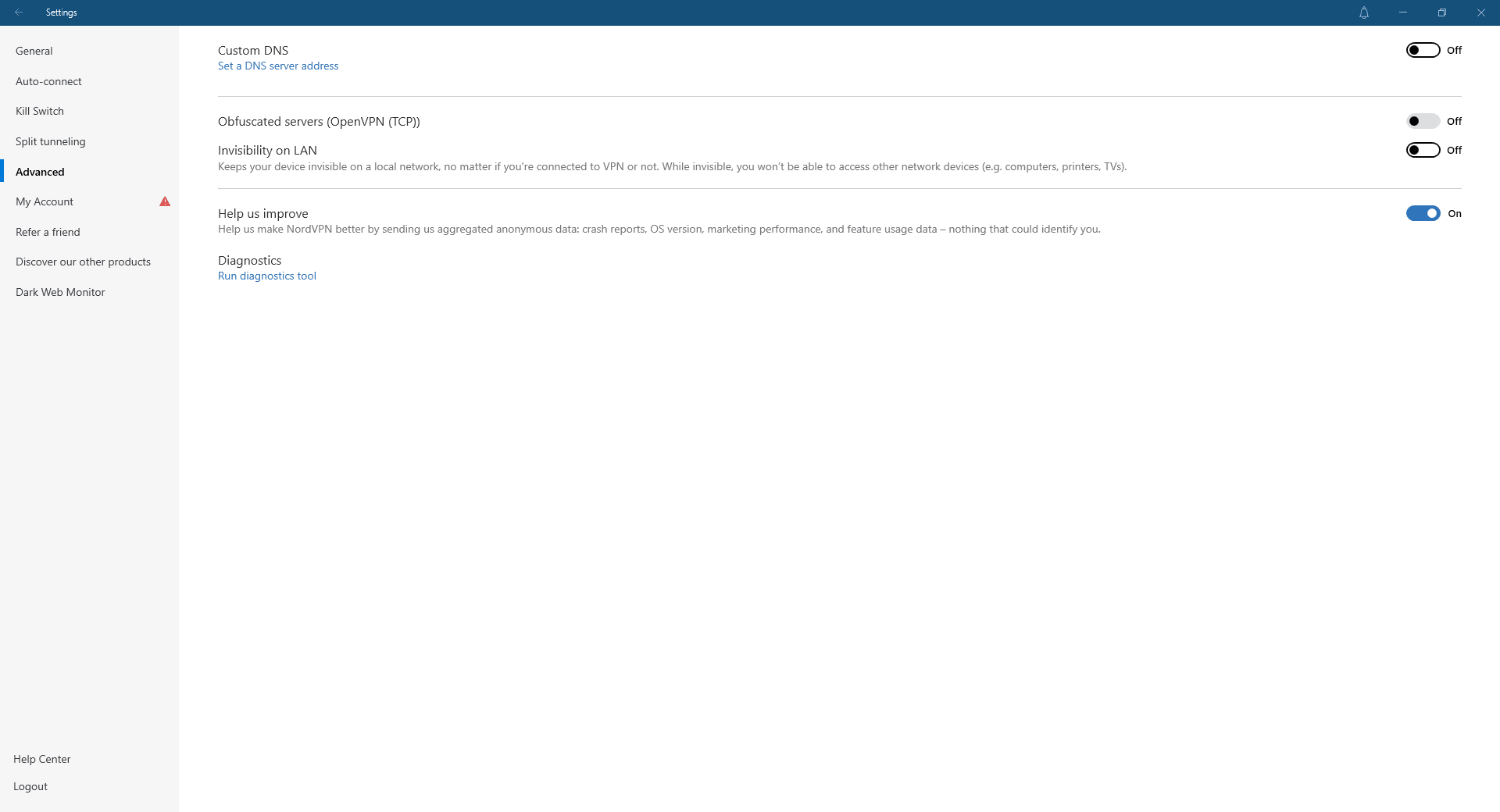A detailed caption for the image could be:

"This screenshot captures the advanced settings page of an application interface. At the top, a thin blue bar labeled 'Settings' spans across the screen, with bell and minimize icons situated on the right side. On the left, a vertical menu displays various options: General, Autocorrect, Kill Switch, Split Tunneling (partially unreadable), Funding, and Advanced. The 'Advanced' section is prominently selected in bold and black, marked by a blue bar to its left. Below 'Advanced,' additional options include My Account, Refer a Friend, Discover Other Projects, and Dark Web Monitor, among others. The main area to the right under the 'Advanced' section reveals detailed features such as Custom DNS with an accompanying description to set a DNS server address, Obfuscated Servers, OpenVPN (TCP), Invisibility on LAN, and Help Us Improve. Some text remains unreadable. Diagnostics options are also present along with a blue button labeled 'Run Diagnostics Tool.' A red triangle alert appears next to 'My Account' in the menu. On the right side of the screenshot, toggle switches indicate the status of various settings. The top three settings (Custom DNS, Obfuscated Servers, and Invisibility on LAN) are toggled off, while the 'Help Us Improve' setting is switched on."